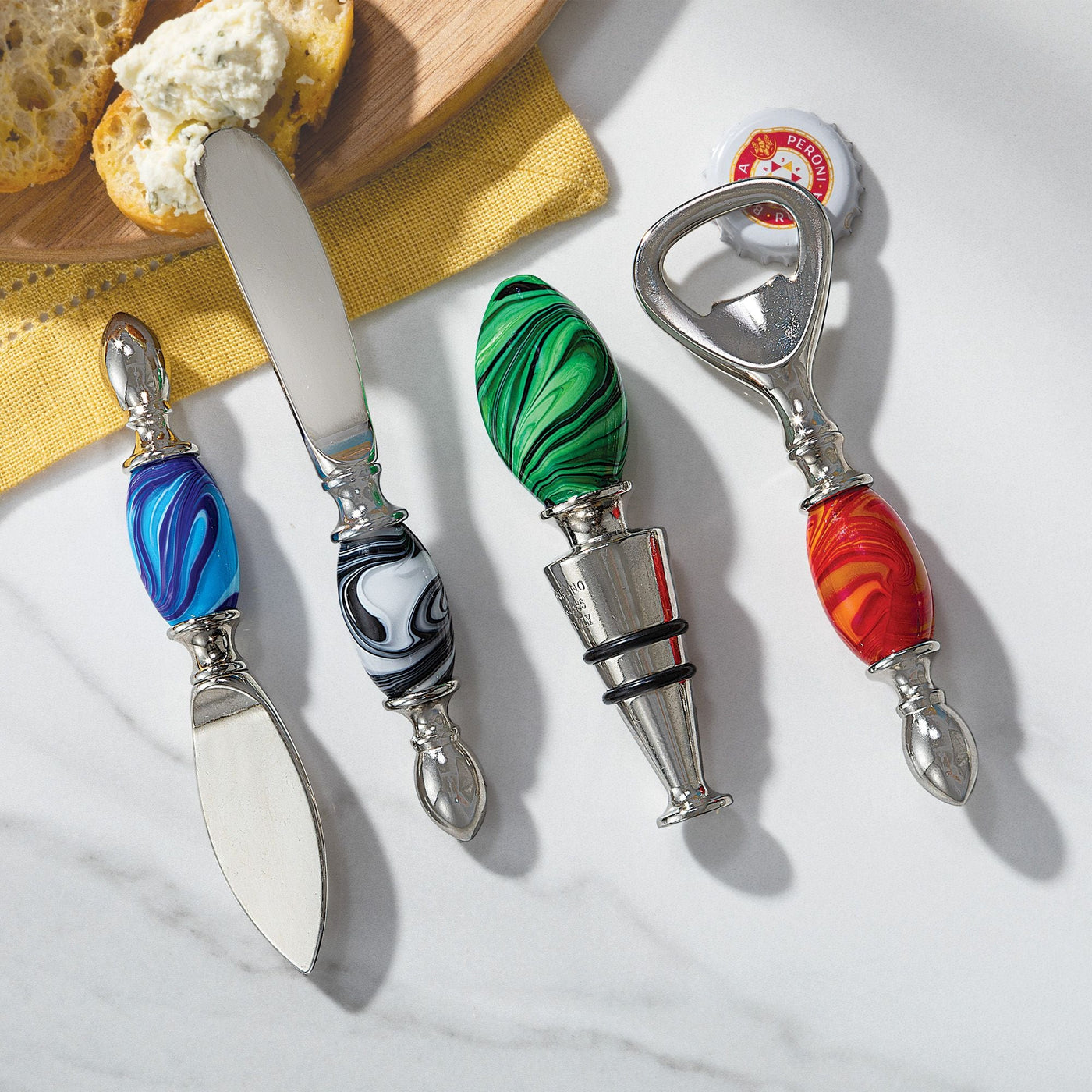In this detailed image, the upper left corner features a yellow napkin and a wooden cheese board with some cheese being applied to a slice of bread. Another slice of bread rests nearby. Dominating the lower part of the image are two cheese cutters and two wine stoppers. The cheese cutter applying cheese to bread has a rounded, gray and black marble handle, while another cutter beneath it boasts a blue and light blue marble handle. Above, a green and black striped wine stopper is displayed alongside a can opener with an ornately swirled red and orange marble handle, with a beer bottle cap positioned beneath it. Scattered across the white table are various corkscrews in blue, silver, green, and red, with the red one also functioning as a bottle opener.